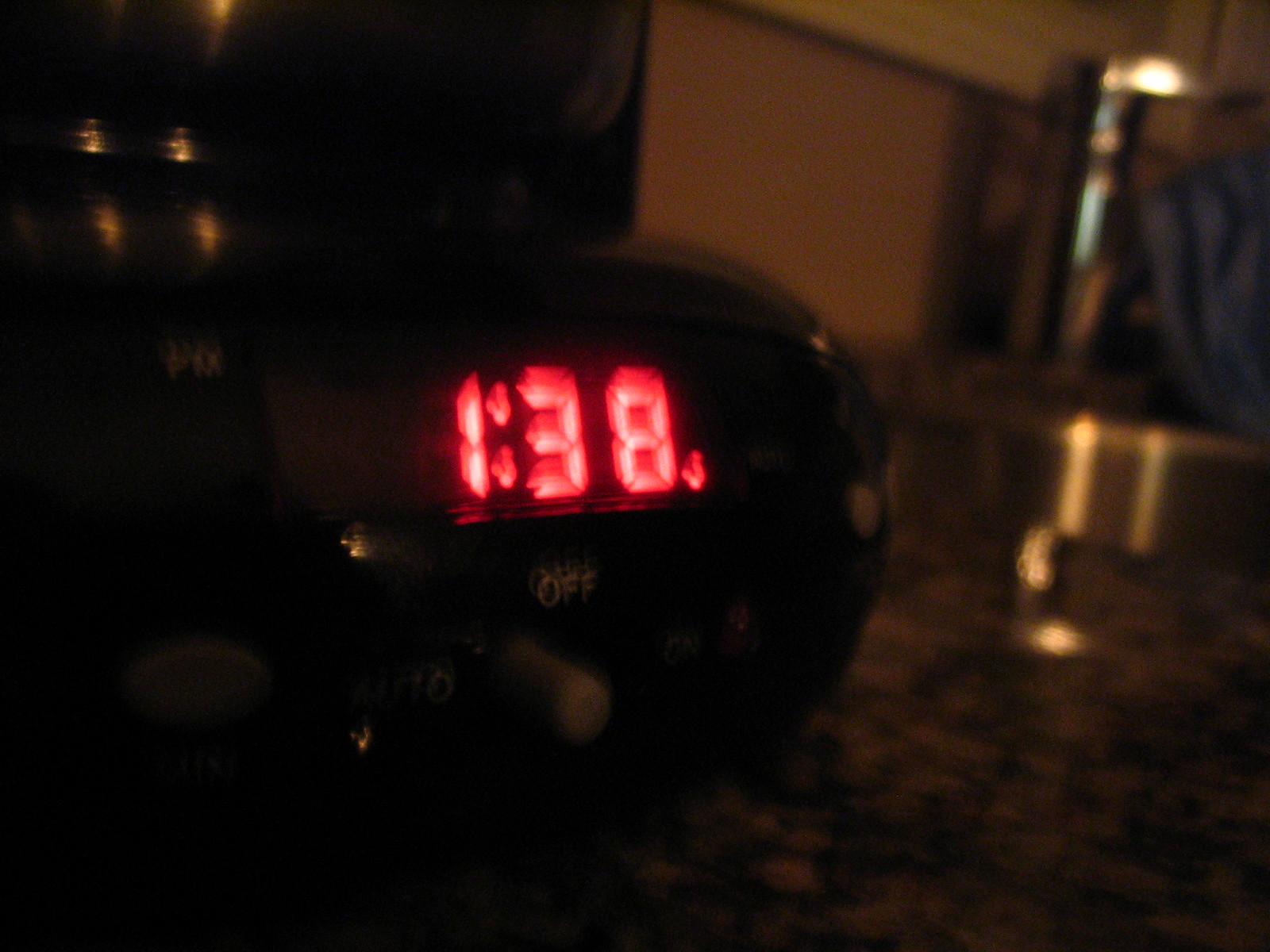A black alarm clock displays the time as 1:38 PM with bright red numbers on its screen. The clock features buttons labeled "Snooze" and "Auto," and an "Off" indicator is visible. The alarm clock is positioned on a nightstand that also holds several containers. At the top edge of the image, the faint outline of a window frame can be seen, suggesting the scene is set in a bedroom.